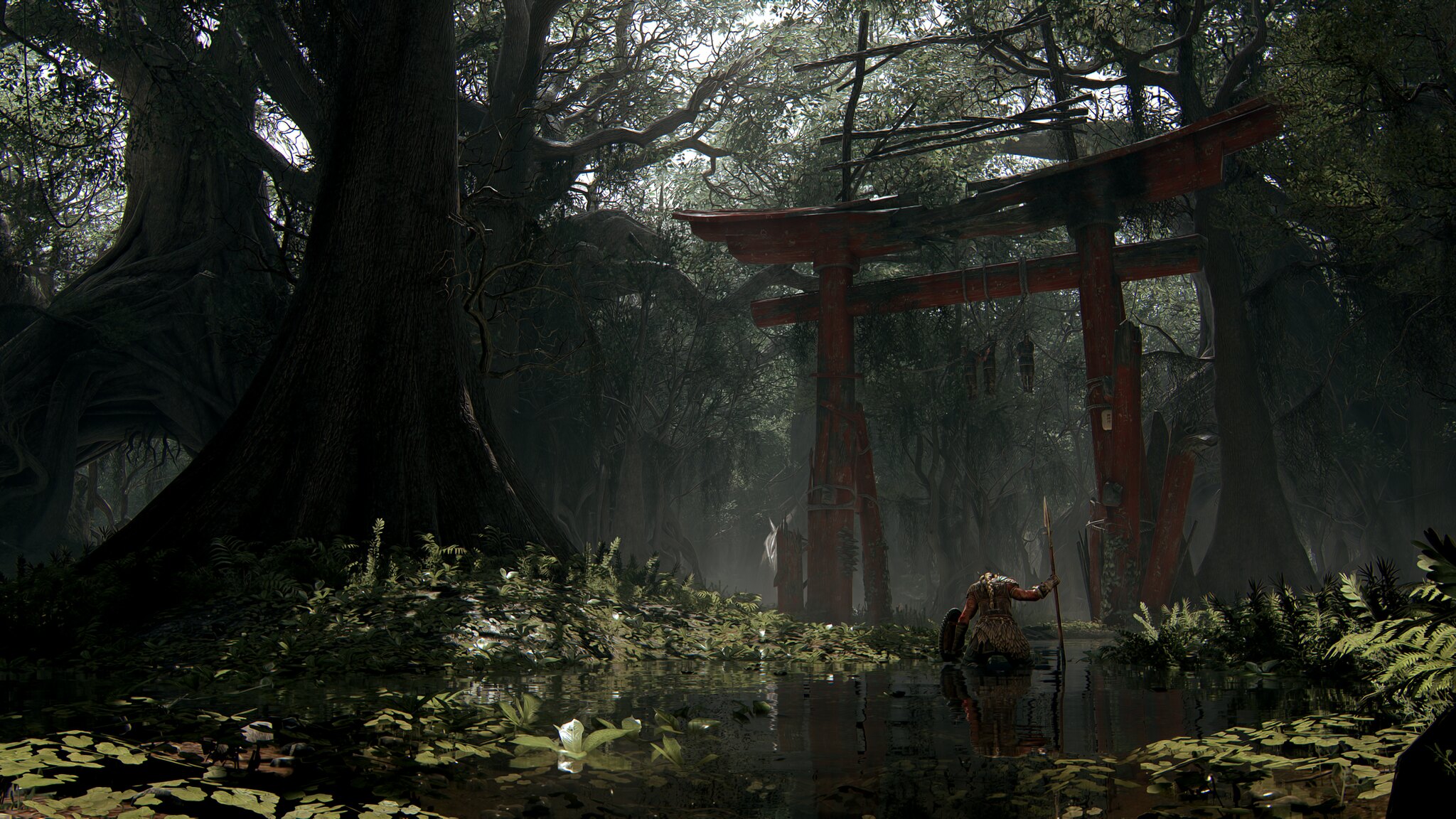In this generated color image, a mystical forest scene unfolds, depicting a swampy area with a tranquil body of water adorned with lily pads and lush, light-green vegetation. Towering, thick tree trunks with large bases and some featuring holes through which glimpses of the white sky can be seen, frame the left side of the image. The right side is almost entirely obscured by dense foliage. Central to the scene, there's a tall, red wooden archway supported by two massive pillars and topped with black sticks, creating a striking contrast with the surrounding greenery. A figure, viewed from the back and dressed in a robe-like garment, wades through the water. The figure, whose head is not visible, carries a long staff with a pointed arrow in one hand and a shield in the other. The serene yet otherworldly ambiance of the setting, combined with the enigmatic character and structure, evokes a sense of a sci-fi or mythical narrative.